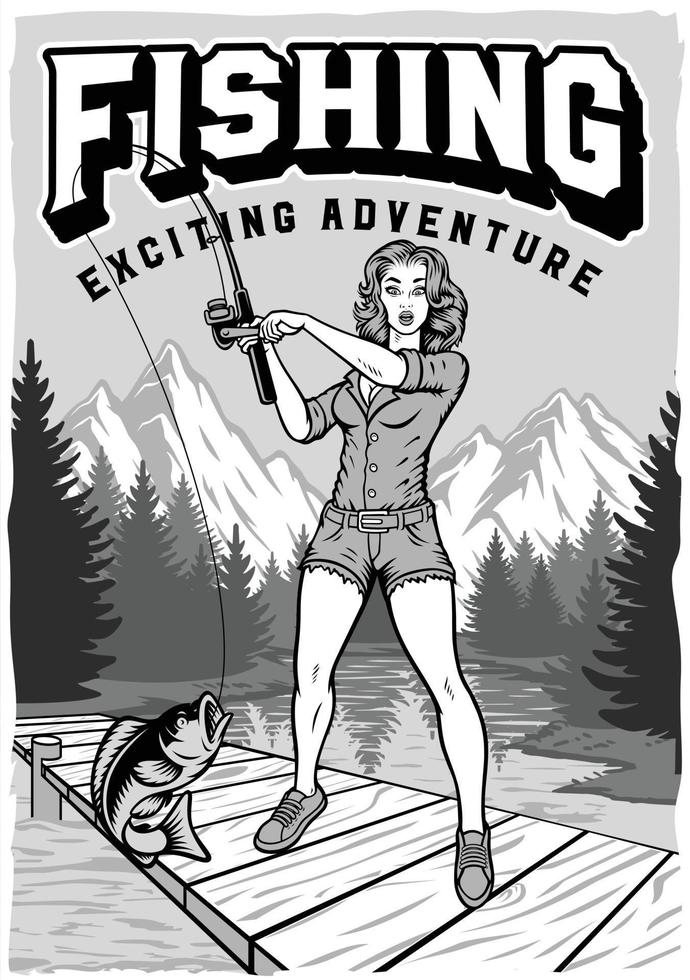The image is a detailed black and white illustration, designed as a modern advertisement for fishing with the captivating tagline "Fishing: Exciting Adventure" prominently displayed at the top in large white letters outlined in black, followed by the same phrase in bold black font beneath it. The focal point of the image is a young, attractive woman standing on a white wooden dock. She is depicted in mid-action, hauling a sizable bass fish up with her black fishing rod. The woman is dressed in a stylish and rugged outfit, featuring a gray button-up mid-length sleeve shirt, gray cutoff shorts with a belt, and gray sneakers or moccasins. She has a surprised expression on her face as she looks at her catch. The background enriches the scene with layers of natural elements: a gray and white lake, pine trees in varying shades of gray and black, and distant wintry mountains, adding a picturesque, adventurous aura to the advertisement.